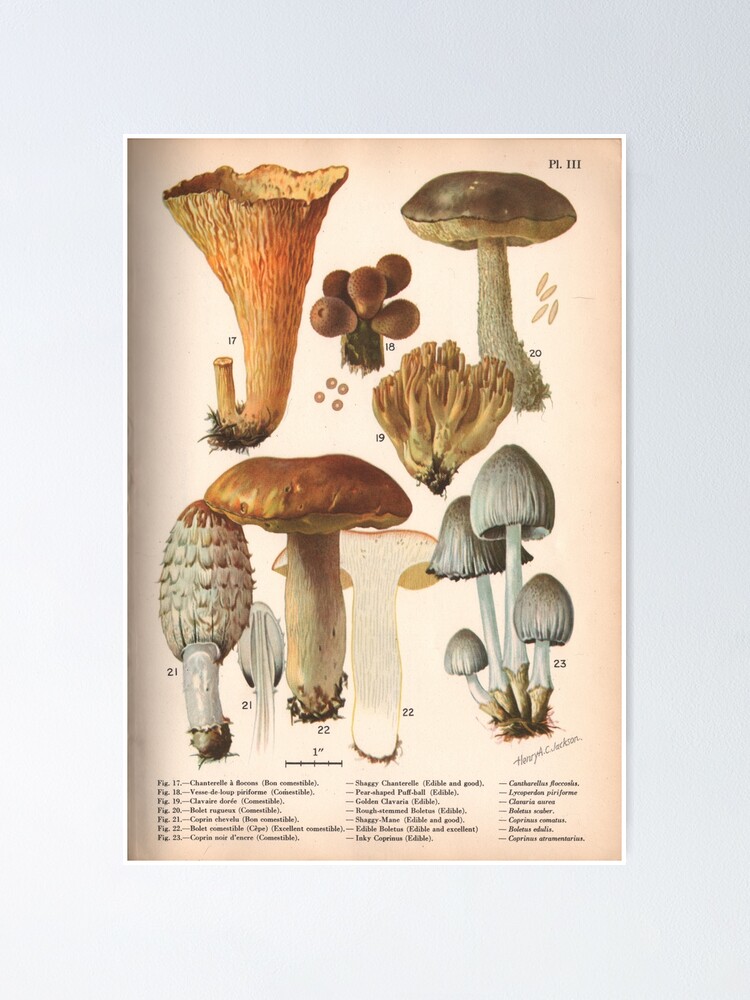This detailed image is an interior page, possibly from a plant or mushroom magazine, specifically page 111 or page 3, featuring an infographic with a white and orange background. The infographic showcases seven different types of mushrooms, each uniquely illustrated and marked with numbers 17 through 23. The drawings are accompanied by their respective names and figure numbers, such as "17. Chantil" and "18. Vestaloupe," suggesting the names might be in French. Notably, mushrooms numbered 21 and 22 include additional images depicting their interiors. Below the illustrations, there is a small bar for size scaling to indicate the relative sizes of the mushrooms. The mushrooms display a variety of caps, including white and brown ones, and all scientific names are presented in clean black lettering, adding a precise and organized touch to the overall infographic.